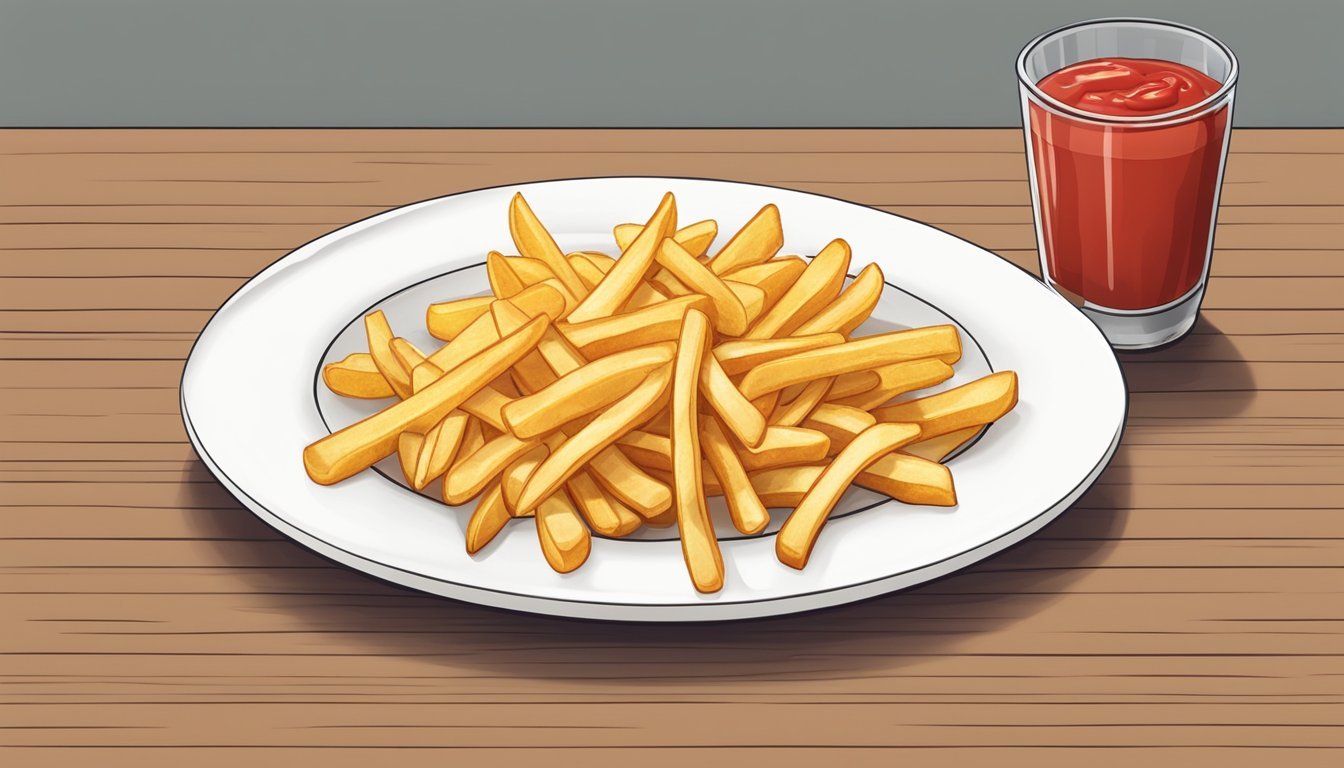The image is an artistic illustration featuring a round white plate with a detailed silver lining on the perimeter and an indentation also outlined in silver. Piled in a pyramid shape on the plate are golden yellow, crispy french fries, enough for at least two people. Adjacent to the plate, on the right side, there is a transparent glass. Notably, this glass appears to be filled with ketchup, although it mimics the appearance of a drink, possibly cola. Both the plate and the glass are positioned on a light to medium brown hardwood table, characterized by parallel grains running horizontally across the image. The background is a minimalist gray, with a distinct strip just beyond the table occupying about one-fifth of the image's height. The overall composition gives a clip-art-like, artistic feel.